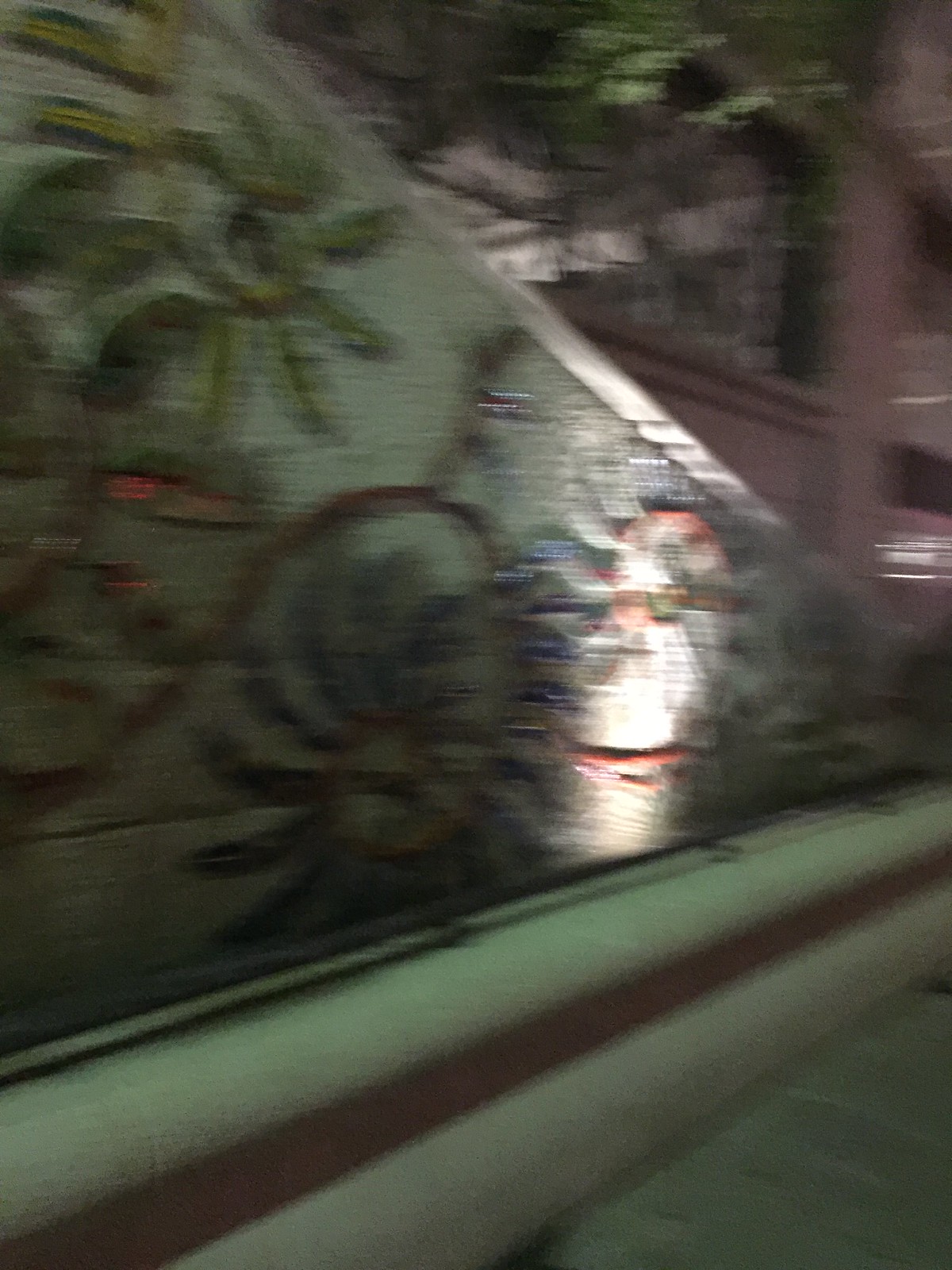The image, taken at night and notably blurry, captures an outdoor scene featuring a large, gray building in the background. This building displays several windows and is partially obscured by trees. In the middle ground, there's a diagonally-shaped wall, likely the side of a staircase or ramp, adorned with colorful floral designs, including brown, yellow, and purple flowers with swirly brown stems. These decorations give the wall a lively appearance despite the image's poor quality. Below this decorative wall, there is a thick guardrail or border that curves in and out, leading to a flat, gray surface, possibly a street or pavement. The overall scene is enhanced by the presence of plants and hints of greenery, making the setting appear vibrant even through the blur and grain. The architectural style and decorative elements suggest a location that could be in Latin America.